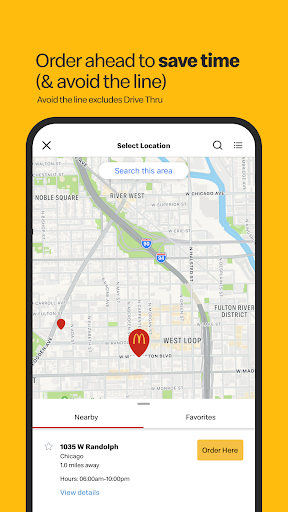The image is part of an advertisement for the McDonald's app, set against a prominent yellow background that embodies the iconic yellowish gold of McDonald's branding. At the top of the image, bold black text reads, "Order ahead to save time," with the phrase "save time" in bold and additional text in parentheses stating, "(and avoid the line)." Beneath this, a note clarifies that "avoid the line" excludes the drive-through.

The central focus of the ad is a detailed screenshot of a smartphone displaying a map, which clearly shows a section of Chicago. Key areas such as West Loop and Fulton River District are prominently marked. A location pin, featuring the McDonald's golden arches, points to the address "1035 West Randolph, Chicago," which is indicated to be one mile away. On the right side of the map, a conspicuous yellow button with black text invites users to "Order Here." This button encourages customers to use the app's convenience features.